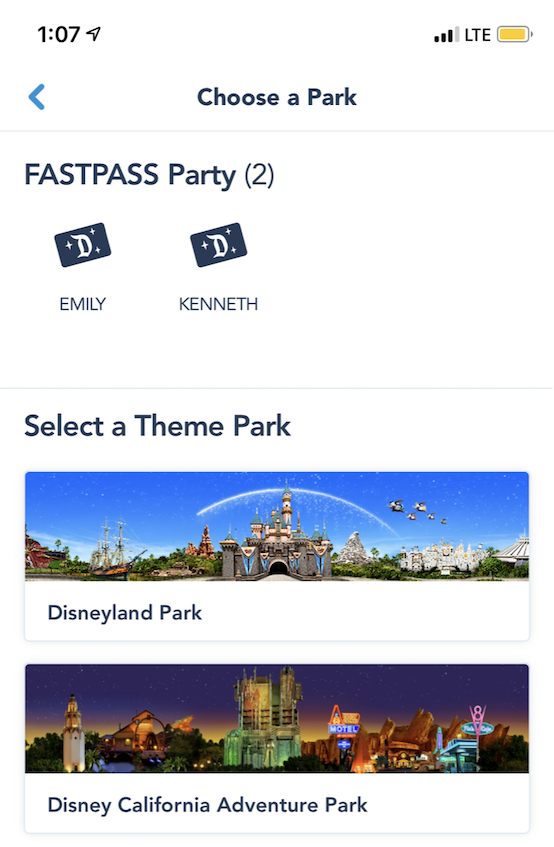A vertical mobile screenshot displaying a clean interface with a white background. In the top-left corner, the time is indicated as 1:07. At the top-right, connectivity status is shown as LTE alongside a nearly full yellow battery icon. Below this, bold blue-black text reads “Choose the Park” with a thin gray horizontal line underneath.

Next, the text “FAST PASS PARTY” is displayed in all caps, followed by “(2)” in parentheses. Two rectangular icons resembling Disney passes appear just below, adorned with a decorative letter "D" and small stars. The left pass is labeled “EMILY” in all caps, while the right one is labeled “KENNETH,” also in all caps.

Another thin gray horizontal line separates the previous section from the bold black text that reads “Select a Theme Park.” Two horizontal rectangular bars are situated below. The top bar showcases an image of Disneyland; it features the iconic grey castle, a blue sky, a white arc, and a pirate ship on the left, with other attractions in the background. Below the image, text on a white strip reads “Disneyland Park.”

The lower bar displays a night-time image of Disney California Adventure Park, highlighted by a well-lit motel sign and other illuminated attractions. Text below this image reads “Disney California Adventure Park.”